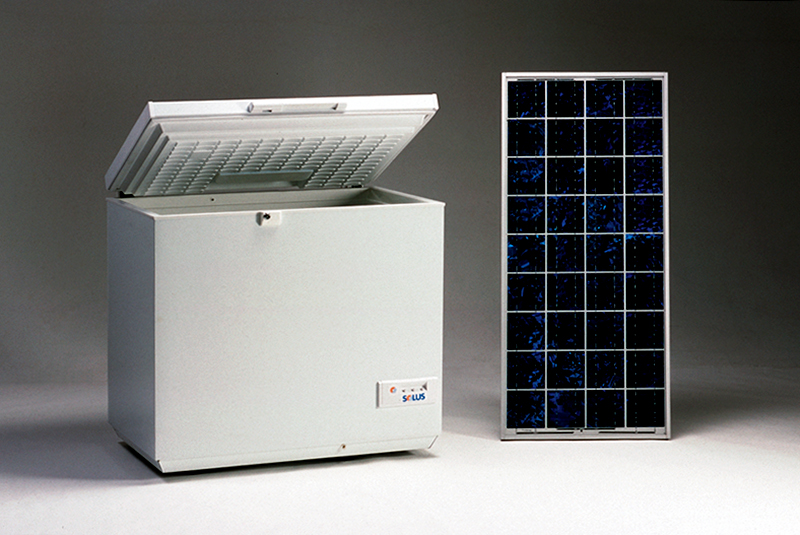The image depicts a scene in a room with a dark gray background and a white floor. On the left side, there is an open mini fridge or small chest freezer with a white lid that opens on a hinge. The interior of the fridge is also white, highlighted by a white latch towards the bottom right corner. The tag on the lower right corner of the fridge reads "SCLUS" with "C" in orange and the other letters in blue. To the right of the fridge, there is a tall, rectangular solar panel with a silver frame. The panel consists of nine pieces of glass in each of its four rows, totaling 36 panes. The surface of the solar panel appears black with blue flecks. Both objects are resting on the white floor, contrasting with the dark tones of the room.